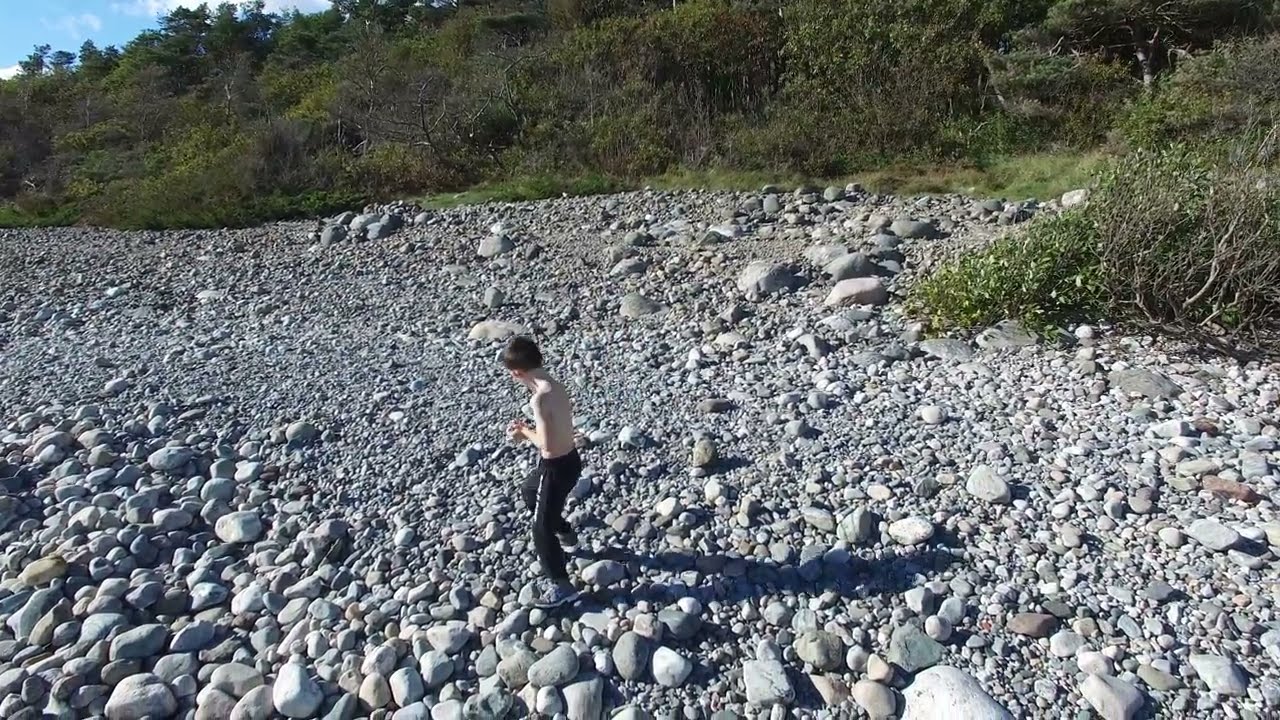The image depicts a serene, rocky shore adjacent to the ocean, under a bright blue sky scattered with a few fluffy clouds. The shoreline features a variety of rocks, ranging from small pebbles to imposing boulders approximately six feet tall. On the right side of the image, a shirtless man in long pants is bent over, examining something of interest among the rocks. The beach's rocky terrain transitions smoothly from large boulders near the water to gravel-sized stones further back. To the right, a verdant hillside with wild grasses, shrubs, and trees gently slopes down toward the shore. The ocean on the left is calm, with gentle waves about a foot tall creating a foamy edge as they lap against the rocks. In the distance, the water is a clear blue, and land is faintly visible on the horizon. The overall scene conveys a peaceful, natural beauty.